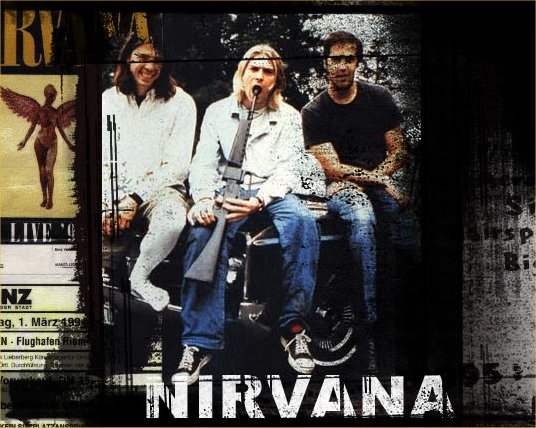The image depicts a dark and intense poster for the band Nirvana, featuring all three members of the band seated atop a large speaker subwoofer, with a rugged, graffiti-like backdrop. Kurt Cobain, positioned centrally, wears a white shirt, blue jeans, and Vans shoes with white shoelaces. Disturbingly, he holds an automatic weapon pointed into his mouth. To Cobain's left, Dave Grohl smiles faintly, dressed in a white shirt and white tights or socks, and looks directly at the viewer. The member on the far right wears a black t-shirt and blue jeans, mirroring Cobain's attire. Both the guy on the right and Cobain appear to be holding guns, contributing to the dark theme. At the bottom of the image, the band's name "NIRVANA" is stenciled in bold white capital letters. To the left of the members, a partial album cover featuring an angel-like figure and fragments of the word "Nirvana" is visible, while the background combines elements of black spray paint and torn posters, evoking a gritty, underground aesthetic. The overall color palette is comprised of black, white, gray, light blue, yellow, orange, tan, and light green tones, adding depth and a somber vibe to the composition.